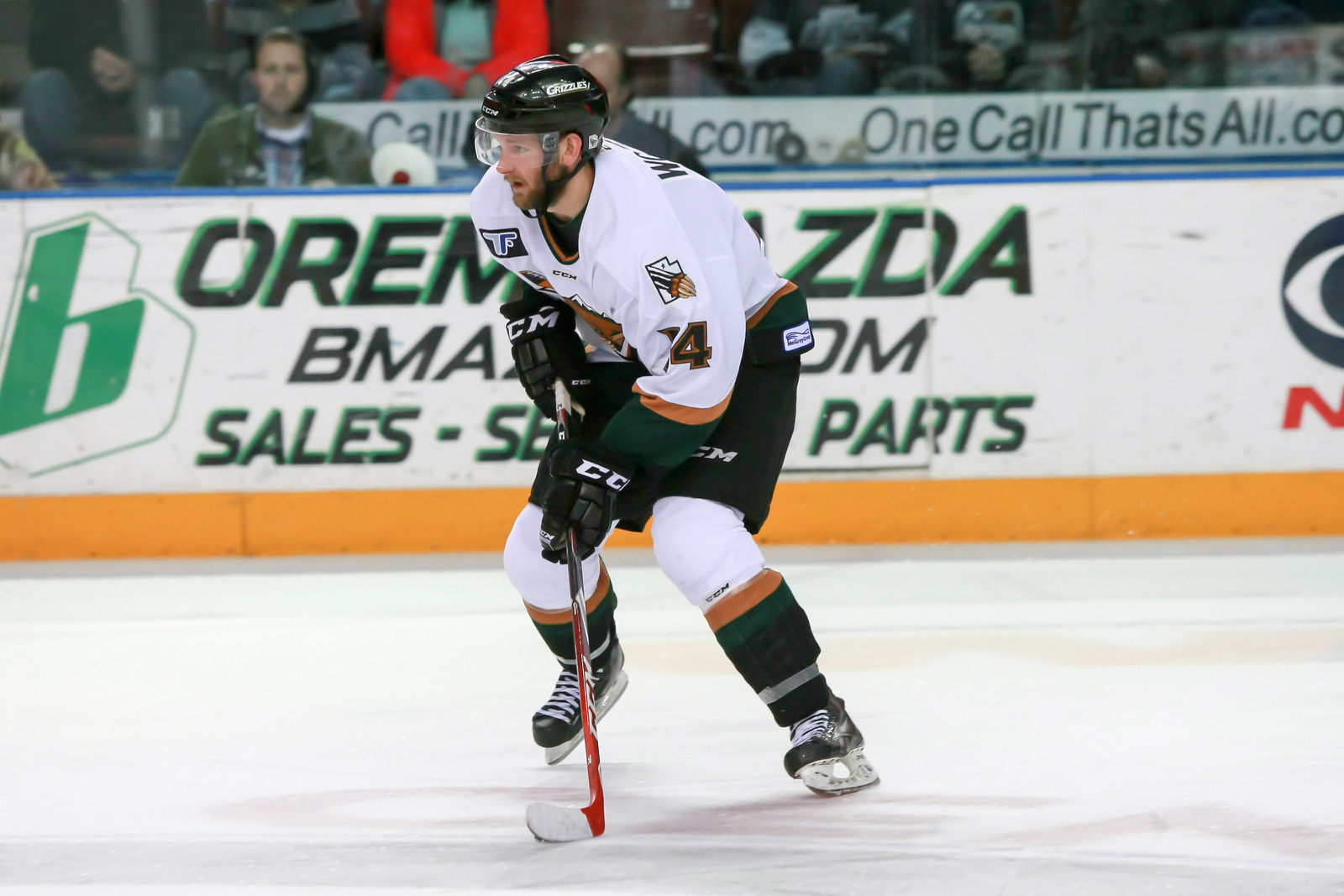A white man, sporting a short beard, is captured on the ice during a hockey game. He wears a black helmet with a clear face shield, a white jersey marked with the number 74, black shorts, white knee guards, black socks over his shins, and black skates with white laces and silver blades. His black gloves with "CC" on them clasp a hockey stick with a red shaft and a white tip, which he holds on the ice in front of him with both hands. He is facing towards the left of the image.

Behind him, a colorful banner is visible with various partial texts due to its obscured placement. The banner presents "OREM" on the left and "ZDA" on the right, followed by "VMA" and "OM" on a lower line, and finally "Sales", "Service", and "Parts" on the third line. A thin blue line runs along the top of the banner, and just above this, spectators can be seen pressed against the plexiglass. Additionally, another banner behind the spectators reads "OneCallThat'sAll.com" on the right side. The white ice rink is evident, marked with the dynamic presence of the hockey player and a backdrop of spectators blending into the scene.